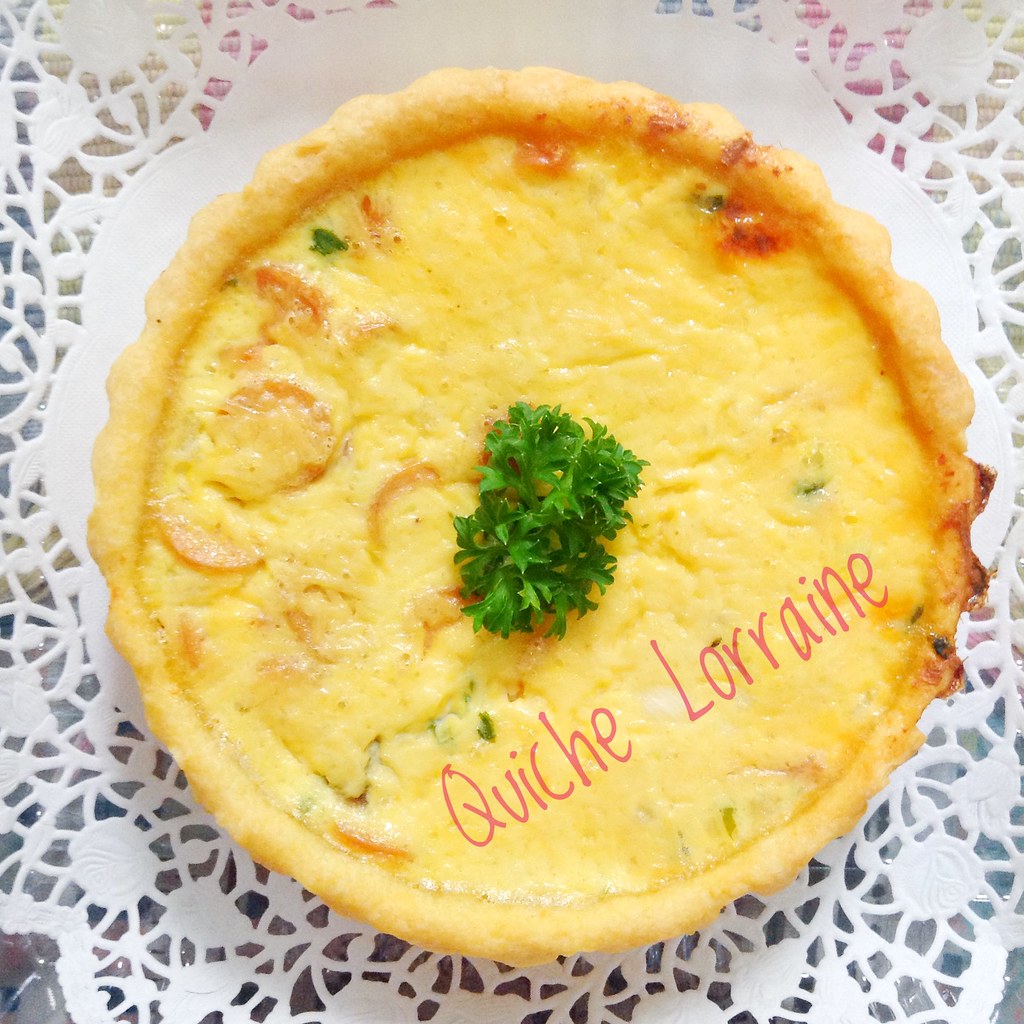This close-up overhead photograph captures a delectable quiche Lorraine perfectly presented on a white, petal-shaped plate, enhancing its elegant appeal. The plate is placed on a delicate white lace doily, with hints of a blue and pink checkered tablecloth subtly peeking through underneath. Dominating the center of the image, the quiche features a golden-brown, crisp crust, indicating it is beautifully baked. The surface of the quiche is smooth, with a rich yellow color accented by caramelized patches of cheese. At the center of this savory dish rests a fresh sprig of parsley, adding a touch of green vibrancy. A soft purple watermark in a marker-style font is visible on the bottom right quadrant of the quiche, subtly adding to the composition. This artistic arrangement makes the classic French dish appear not only appetizing but also visually captivating.